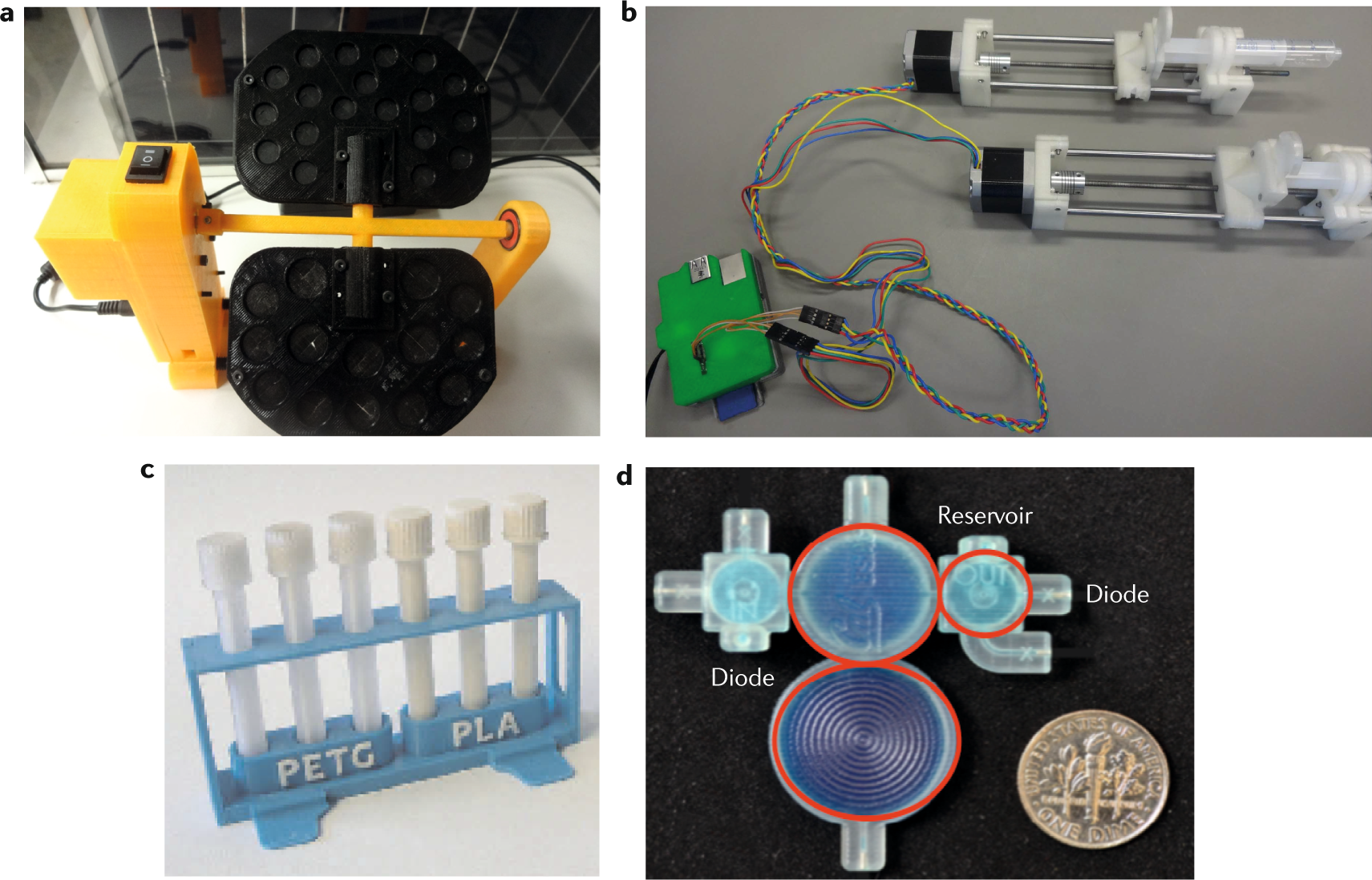The image comprises four separate sub-images labeled A, B, C, and D, arranged in a 2x2 grid. 

- **Image A (Top Left)**: Displays a robotic-like mechanism placed on a white surface. The main body is yellow, featuring a prominent switch and protruding wires, flanked by two wide, black, arm-like paddles with circular holes, reminiscent of industrial equipment.
  
- **Image B (Top Right)**: Features electrical components connected by wires. Central to this image is an insulated wire linked to two metallic rods encased in white plastic. These are connected to a small green cuboidal box situated in the bottom left corner of the image. The background color is gray.
  
- **Image C (Bottom Left)**: Shows scientific vials, which are white and arranged in a blue container. The container is labeled with "P-E-T-G-P-L-A," and the background is light gray.
  
- **Image D (Bottom Right)**: Depicts a detailed diagram labeled "diode, reservoir, and diode," accompanied by a silver coin, illustrating the size of the components. The machine-like diagram has several pipes and annotated lines, set against a black background.

The entire composite image has a white outer background framing these individual pictures.